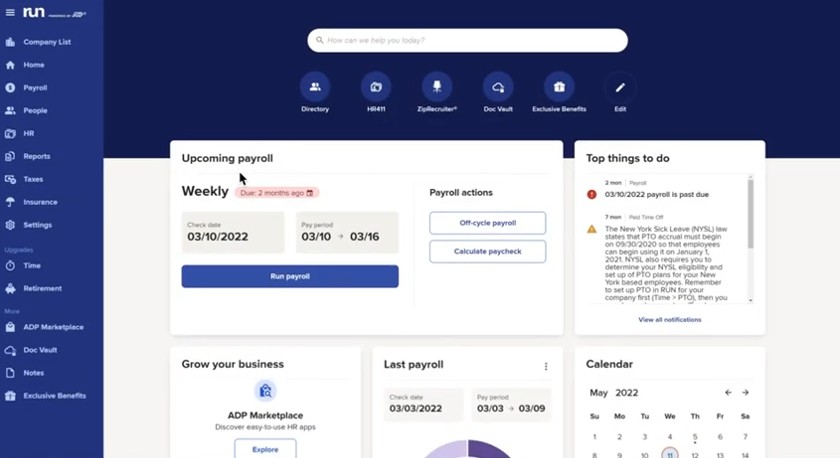This image depicts an admin panel for a site called RUN, specifically focused on payroll management. On the left side of the interface, there's a prominent logo followed by a comprehensive vertical menu. At the top of this menu is the word "RUN." The menu contains multiple sections, each accompanied by an icon: Company List, Home, Payroll, People, HR Reports, Taxes, Insurance, Settings, Time, Retirement, ADP Marketplace, Doc Vault, Notes, and Exclusive Benefits. The background of this menu is light blue.

Across the top of the admin panel is a darker blue horizontal menu with several features. There's a search bar featuring the term "Directory HR 411." Other visible elements include possibly "ZipRecruiter," "Doc Vault," and "Exclusive Benefits," all of which are blurry. There's also an option for editing.

The main workspace of the panel displays the upcoming payroll details. A prominent red notification indicates that the payroll is overdue by two months, with a check date of March 10, 2022, and a pay period spanning from March 10 to March 16. Below this section, there's a "RUN Payroll" button along with options like "Payroll Actions," "Off-Cycle Payroll," and "Calculate Paycheck."

In the lower part of the image, there are various reminders and a to-do list, such as "Payrolls Past Due" and additional notes. A calendar is partially visible with text mentioning "Grow Your Business," "Last Payroll," and "Calendar." A circular graph is also present, though its details are indistinguishable.